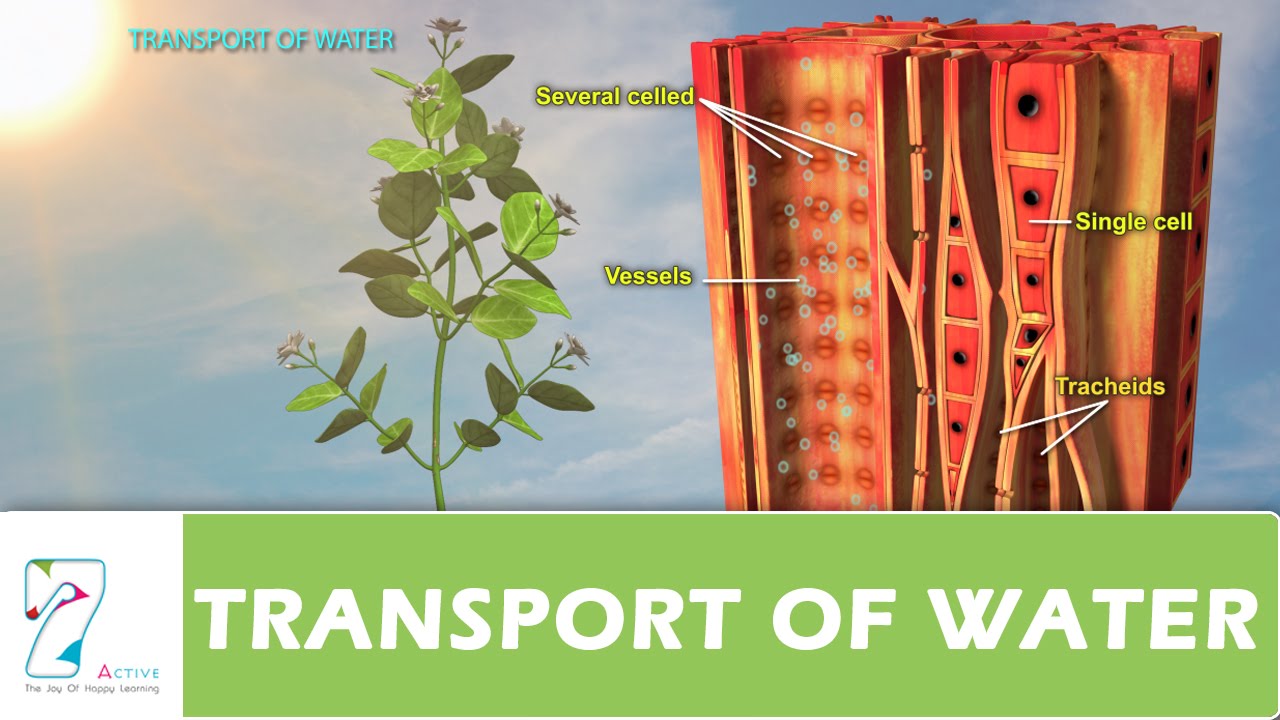This educational image from Seven Active illustrates the transport of water within a plant. At the center, a green plant with a couple of stems and leaves showcases a magnified view of its internal structure on the right side, depicted in red and orange colors. This detailed diagram features several celled vessels, single cells, and tracheids, with vertical columns and black dots highlighting the internal workings. To the left of the plant, a glowing yellow and orange sun is visible, with the text "transport of water" next to it. The image has a sky-like blue background that sets off the various elements. At the bottom, there is a bright green rectangle with white sans serif font that reads "transport of water" in a large size. To the left of this green box is the Seven Active logo which states, "active the joy of happy learning," and includes a distinctive turquoise number seven with a white interior and accents of lime green, magenta, and turquoise blue.